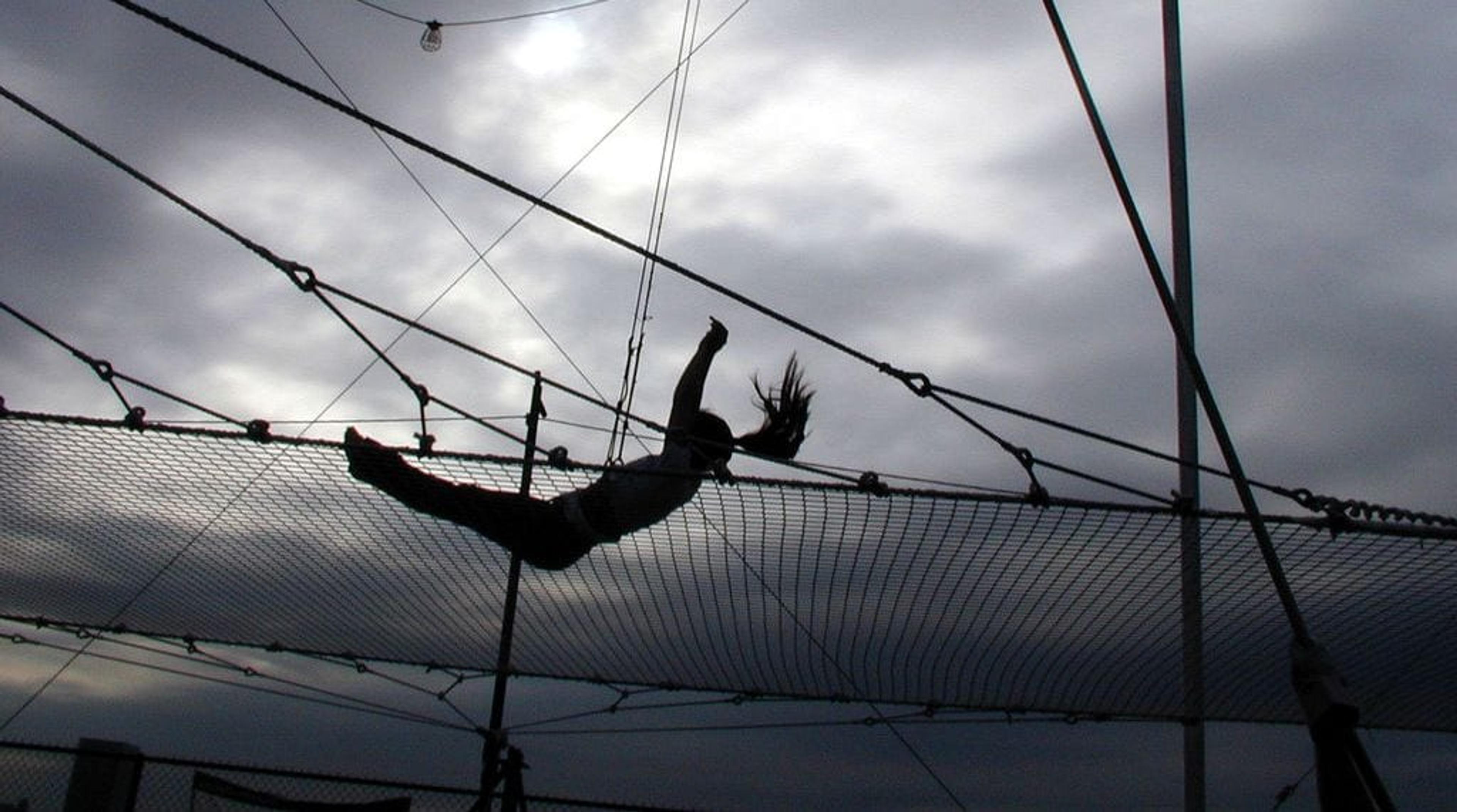This is a shadowy, monochromatic photograph taken from the ground looking up at a suspended trampoline, most likely at dusk. The sky in the background is a very grayish violet, with light patches breaking through the clouds. Dominating the scene is the silhouette of a girl with a long black ponytail caught in mid-bounce, her body forming a flattened V shape. She appears in profile with one arm raised and her legs and feet pointed together, giving a dynamic sense of motion as she flies through the air. The trampoline's black netting and crisscrossing cords are sharply outlined, as are the supporting poles and carabiners that connect it to an unseen structure. The photo, rich in shades of gray and black, captures the energy and flight of the moment against a moody sky.